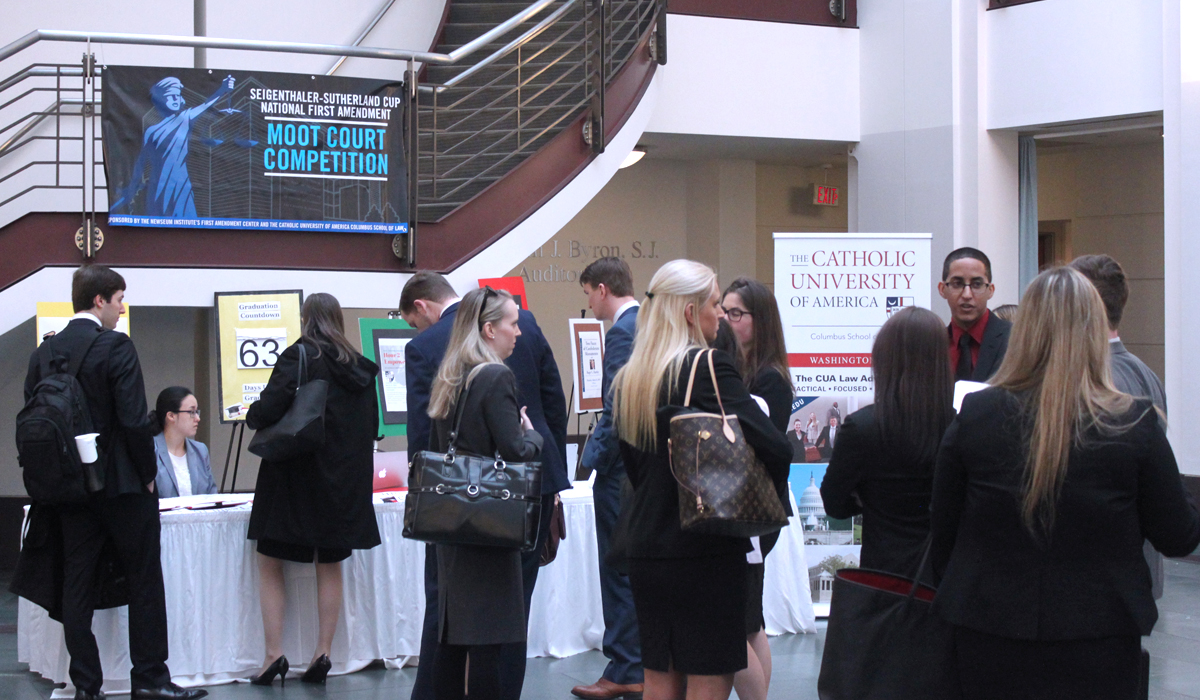This photograph captures a bustling scene inside a spacious hall at the Catholic University of America, where attendees are gathering for an important event. Predominately dressed in professional black attire, including black coats, pants, and skirts, many of the women are seen with handbags slung over their shoulders. A long table draped with a pristine white tablecloth serves as a check-in counter at the front, where people are submitting applications or registering for the event. Behind this counter, individuals are seated, assisting with the process.

Prominently featured on the staircase in the upper left corner is a large banner announcing the "Segenthaler Sutherland Cup National First Amendment Moot Court Competition," accompanied by an image of the scales of justice. Below this visual and the title, the words "Moot Court Competition" stand out in blue letters. 

Participants in line at the desk include a man in a black suit with a backpack and a woman with a black coat and handbag. In the right corner, three women in black coats, one carrying a brown and yellow handbag, are engaged in conversation with a bespectacled man in a black suit, red shirt, and black tie. Additionally, a standalone board sign nearby bears the name "Catholic University of America," contributing to the organized atmosphere of the event. The walls of the hall are primarily white, with some sections in light brown, contributing to the overall elegant and formal setting.